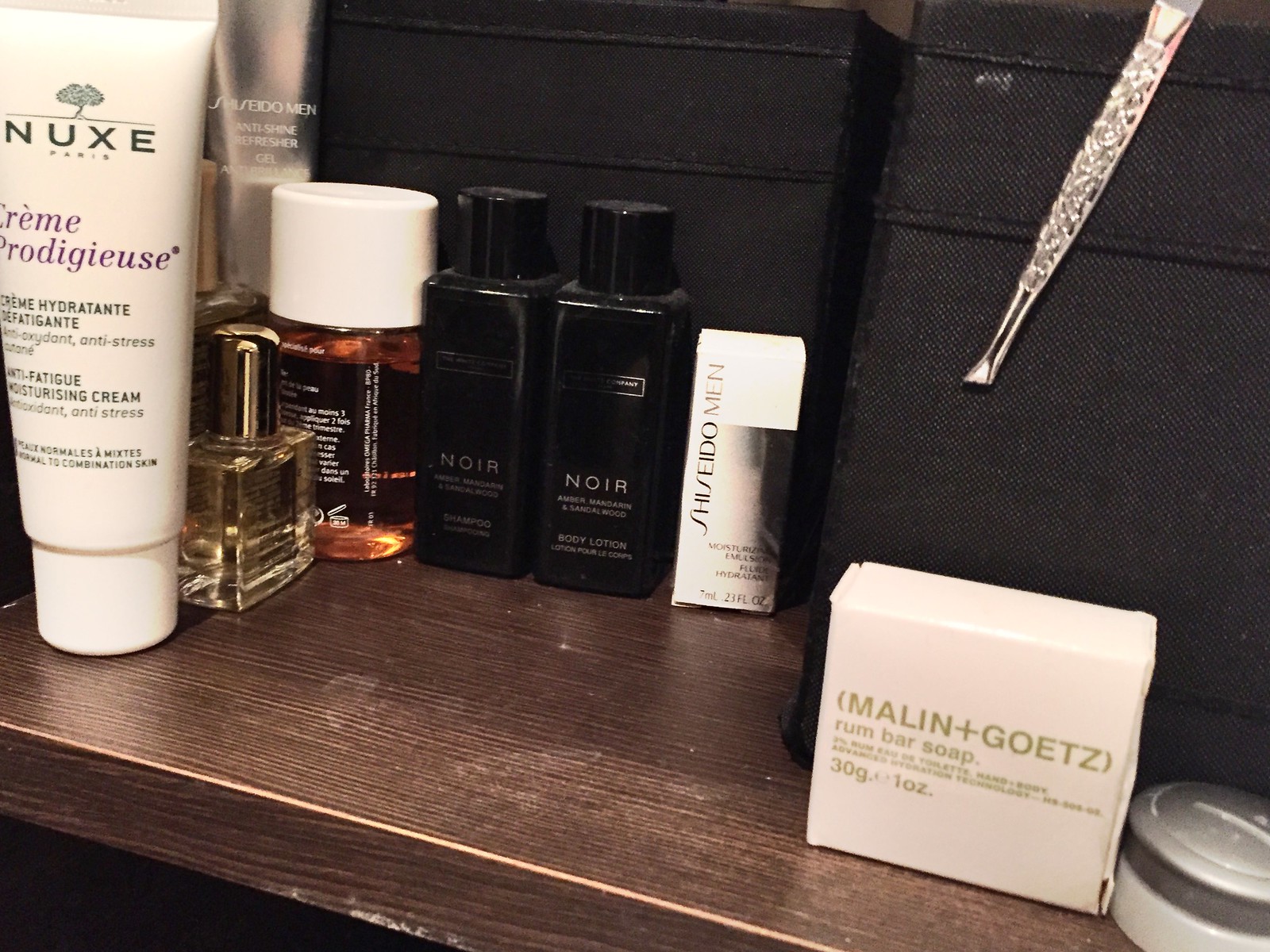The image features a meticulously arranged collection of men's grooming products on a wooden table. On the left side, prominently displayed is a product labeled "Nuxe Prodigieux Anti-Fatigue Moisturizing Cream." Next to it is a clear glass bottle with a golden cap. Beside this, there is a bronze-colored bottle with a white cap. Centrally located are two sleek black "Noir" bottles. Toward the middle right, a small white rectangular box is visible. In the top right corner, a pair of grooming clippers or pliers can be seen. In the bottom right corner, "Malin + Goetz Rum Bar Soap" is noted. The background is dominated by several black boxes on the right and middle areas. At the back left, a men's shampoo product is partially visible. Also, a tiny petroleum-based cream rests on the bottom right corner. The bottom left corner has a black void, creating a contrast with the rest of the detailed display of men's fashion and grooming goods.